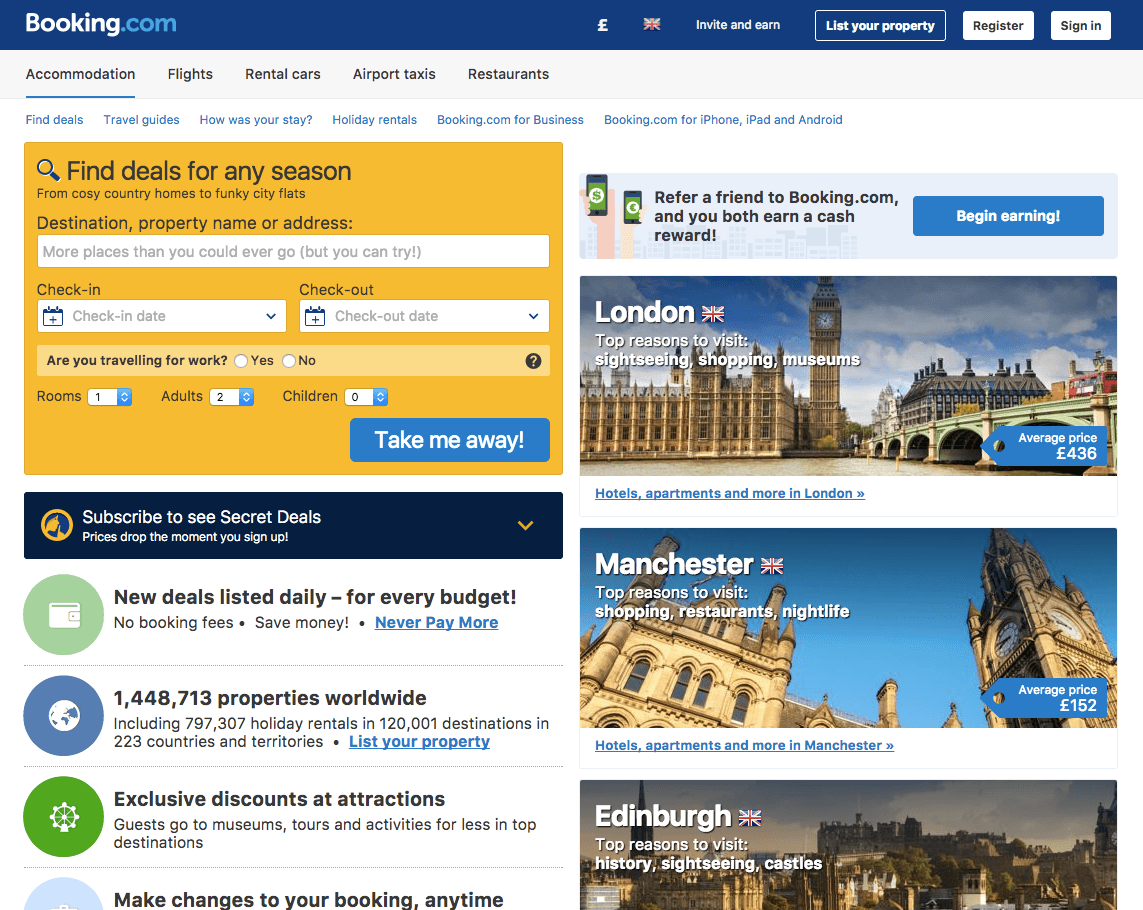This image is a detailed screenshot of the Booking.com website interface. At the top, a blue banner prominently displays the Booking.com logo on the left. On the right side of the banner, there's a box with options for "List your property," "Register," and "Sign in."

Below the banner, the background switches to white, featuring black tabs for various services such as Accommodation, Flights, Rental Cars, Airport Taxis, and Restaurants. The Accommodation tab is currently selected. Directly beneath in blue, there are links for "Find Deals," "Travel Guides," "How was your stay?," "Rental Holidays," "Booking.com for Business," and "Booking.com for iPhone, iPad, and Android."

On the left side of the page, an orange box highlights text promoting deals for any season, ranging from cozy country homes to funky city flats. It includes fields for entering a destination, property name, or address, with corresponding input boxes for the check-in date, checkout date, work travel indication, room number, and number of adults and children. There's also a prominent "Take me away" button to initiate the search.

Below this, another area encourages users to subscribe to see secret deals, promoting new deals listed daily for every budget, access to 1,448,713 properties worldwide, exclusive discounts at attractions, and the ability to make changes to bookings anytime.

To the right, there are three featured photos of popular destinations with captions:
1. London: Top reasons to visit include sightseeing, shopping, and museums, with an average price of £436.
2. Manchester: Top reasons to visit include shopping, restaurants, and nightlife, with an average price of £152.
3. Edinburgh: Top reasons to visit include history, sightseeing, and castles.

Each section is meticulously designed to entice and inform prospective travelers of the robust offerings available on the platform.